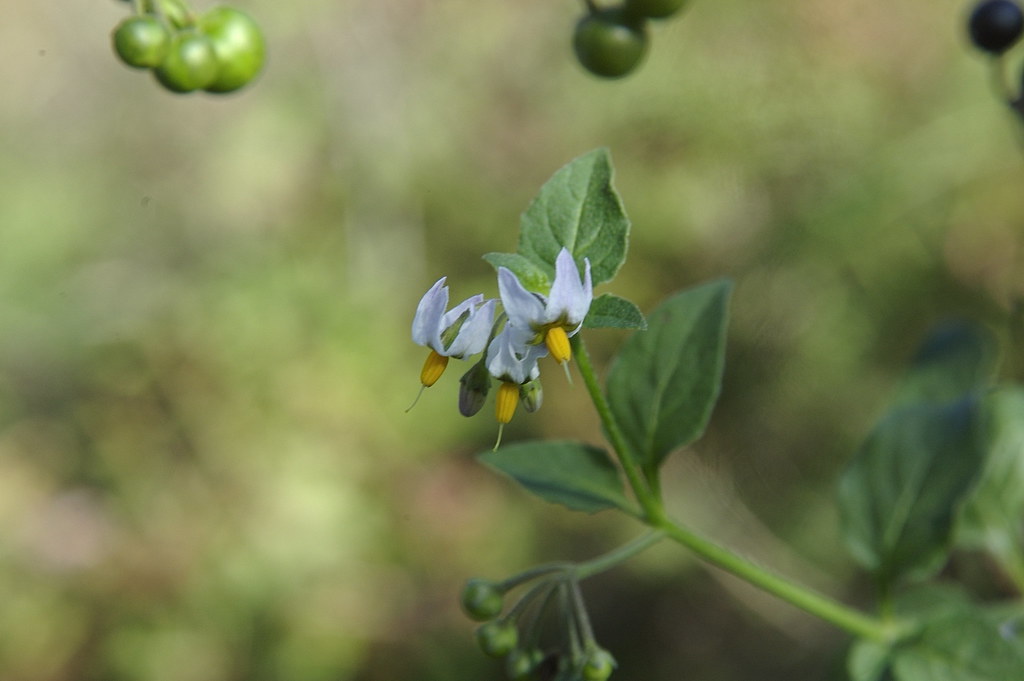This photograph captures a close-up of a black nightshade plant branch. The image focuses on three white flowers, each emerging from a green stem. The flowers hang downward, with petals curving upwards towards the stem, resembling peeled corn husks. Each flower has a central yellow pistil with a slender white filament extending from it, indicating the pollen area. Surrounding the flowers are small, teardrop-shaped green leaves, and scattered throughout the image are small green berries. The background is a blurry green, emphasizing the sharp details of the plant and its various elements.